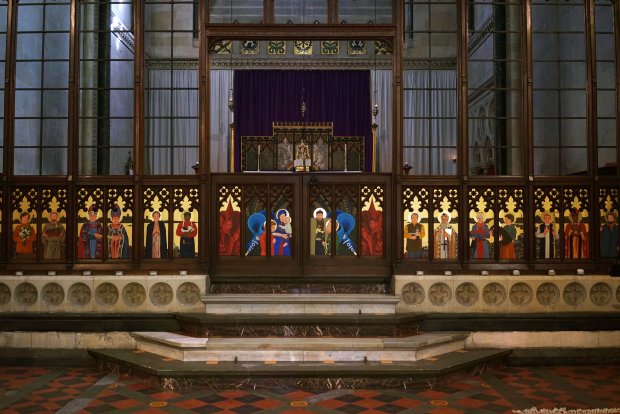The image depicts the interior of an ornate, old Eastern Orthodox church, focusing on the front altar area. It showcases a half-wooden wall adorned with intricate paintings of people in ceremonial attire, prominently featuring dark wood tones and a bright yellow background that appears to glow, possibly due to backlighting. The half-wall in the center includes a half-door and is flanked by open wooden structures stretching from top to bottom. Prominently colored stained glass images, framed within detailed woodwork, decorate the area, primarily in hues of yellow, blue, and green. These images, likely icons, exhibit various figures holding religious artifacts. The altar, raised by two wide marble steps, has a floor adorned with red, black, and grey designs, leading toward the pulpit. Behind the altar, navy or black curtains take center stage, surrounded by long white curtains on both sides. The setting is slightly illuminated by a light situated at the left corner of the image, enhancing the rich, ceremonial atmosphere.